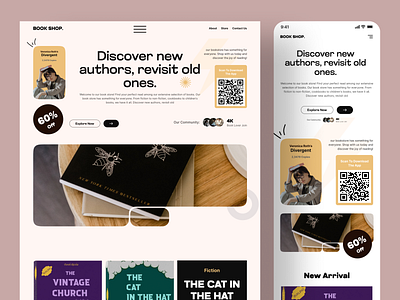Here's a detailed and cleaned-up caption for the described image:

---

The image captures a promotional flyer laid out on a hardwood floor. The flyer features an eye-catching heading that reads "Discover New Authors, Revisit Old Ones." Prominently displayed is a QR code next to a vintage illustration of a person steering what appears to be a wagon wheel. The flyer also advertises a "60% Off" discount and showcases an old-style passport on top of the brown paper. Below, there are smaller graphics including a playful illustration of the Cat in the Hat and another titled "Vintage Church." Adjacent to the larger flyer is a smaller, bookmark-sized version that echoes the same promotional message, designed to hang on a doorknob, reiterating the call to discover new authors and revisit beloved ones.

---